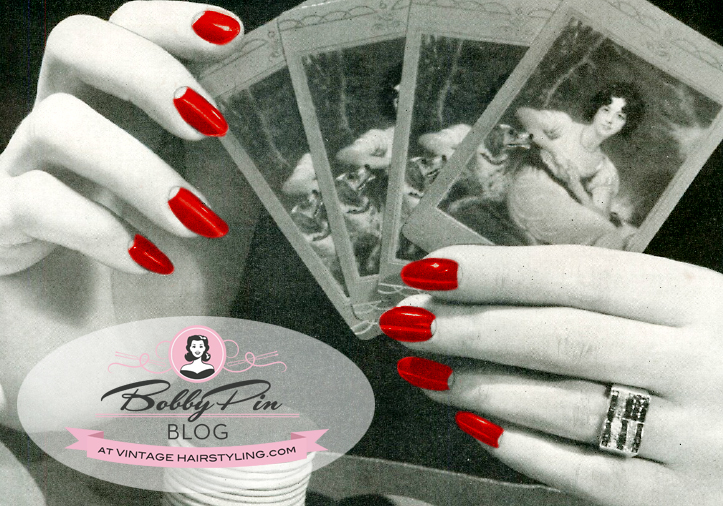The horizontally aligned rectangular image is primarily in black and white, with select splashes of color for emphasis. It features a pair of closely positioned hands, one showing the back with dark red nail polish, and the other displaying the front, also with similarly bright nail polish. Both hands are holding four black and white cards, each depicting a seated woman with black hair and a dog beside her.

In the lower left corner of the image, there's a grayish-brown oval-shaped area reading "Bobby Pin Blog" at its center. Above this oval, a pink-shaded circle contains a black and white illustration of a woman's head with pink squiggly lines emanating from it. Additionally, beneath the oval, a pink rectangular banner with black text reads "at vintagehairstyling.com."

Aside from the vivid red nail polish, the prominent pink elements of the logo, and the banner, the rest of the image retains a monochromatic scheme, creating a striking contrast.